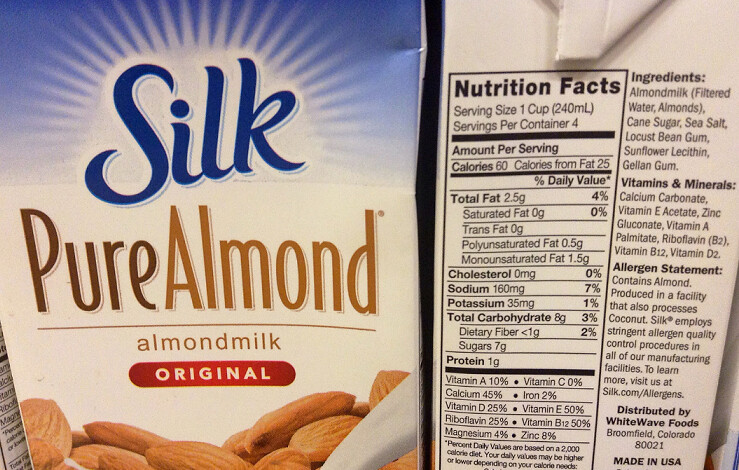This color photograph captures two Silk Pure Almond milk cartons, prominently featuring the logo and various details on the packaging. The logo, scripted in dark blue cursive, evokes sun rays emanating against a deep blue background, suggesting a rising sun. Below this logo, "Pure Almond" appears in a gradient of dark brown transitioning to light brown, leading into "Almond Milk" in a matching brown hue. The label also includes a distinct red, rounded rectangle with "Original" written in bold white letters. At the bottom of the carton, an image showcases a generous heap of almonds with almond milk cascading over them from the side. The photograph further highlights the side panel of the carton, which is white, featuring extensive nutritional information, ingredient list, vitamins and minerals, and an allergen statement all printed in black text. Key nutritional details include per serving: 60 calories, 2.5 grams of total fat, 0 grams of saturated and trans fat, 0 milligrams of cholesterol, and 160 milligrams of sodium. The ingredient list comprises almond milk (filtered water, almonds), cane sugar, sea salt, locust bean gum, sunflower lecithin, and gellan gum.